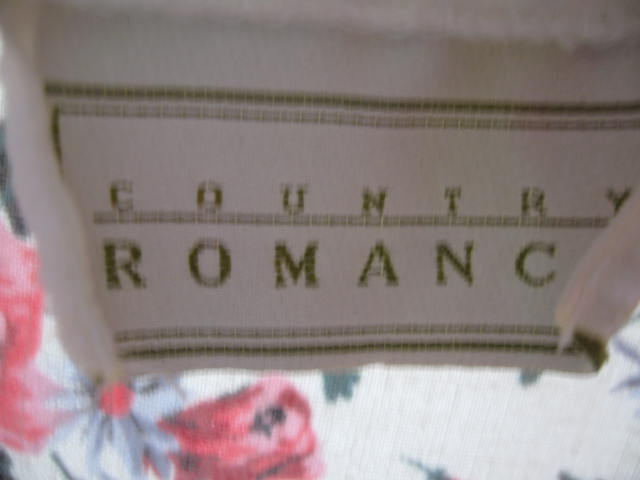In this photograph, a white towel is prominently featured, hanging down from a curtain rod or another horizontal surface. The towel's lower corners are slightly curled forward, partially obscuring the main body of the fabric. The towel is adorned with dull green embroidery or printing, forming a rectangular, bordered shape with the words "Country Romance" in the center. Notably, the 'E' in "Romance" is partially hidden by one of the curled edges of the towel. The photograph itself is low-resolution and somewhat blurry, making the details less distinct. The background features fabric with a pattern of red and grey printed flowers, predominantly on the left side, while the right side appears mostly white.